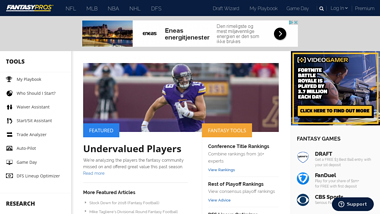At first glance, this appears to be a screenshot from a sports website dedicated to football, specifically one focusing on fantasy sports. The website is identified as "FantasyPros" at the top. A navigation menu features various sports-related categories including NFL, MLB, NBA, NHL, and DFS (Daily Fantasy Sports). 

The available sections within the website likely include options to explore draft advice and tools, with subsection labels hinting at specific functionalities such as "Draft Tools" and "My Playbook." Additionally, the menu offers links named "Game Day" and "My Tools," along with options for logging in and accessing premium content.

Several titles are discernible on the page despite some text being blurry. Notable headlines include "Underappreciated Players," "Most Featured Articles," "Top Player Rankings," and "Bankage Rankings." These articles presumably delve into player analysis, strategy, and rankings within fantasy sports.

At the center of the screenshot, there is an image of a football player, who appears to be from LSU (Louisiana State University) based on the purple uniform accented with a gold or orange stripe on the sleeve. 

To the left, there is a menu of tools, listing options like "My Playback," "What Should I Search," "Game Day," and other functionalities designed to assist users in managing their fantasy sports teams.

Overall, the screenshot indicates a highly detailed, resource-rich platform for fantasy sports enthusiasts.